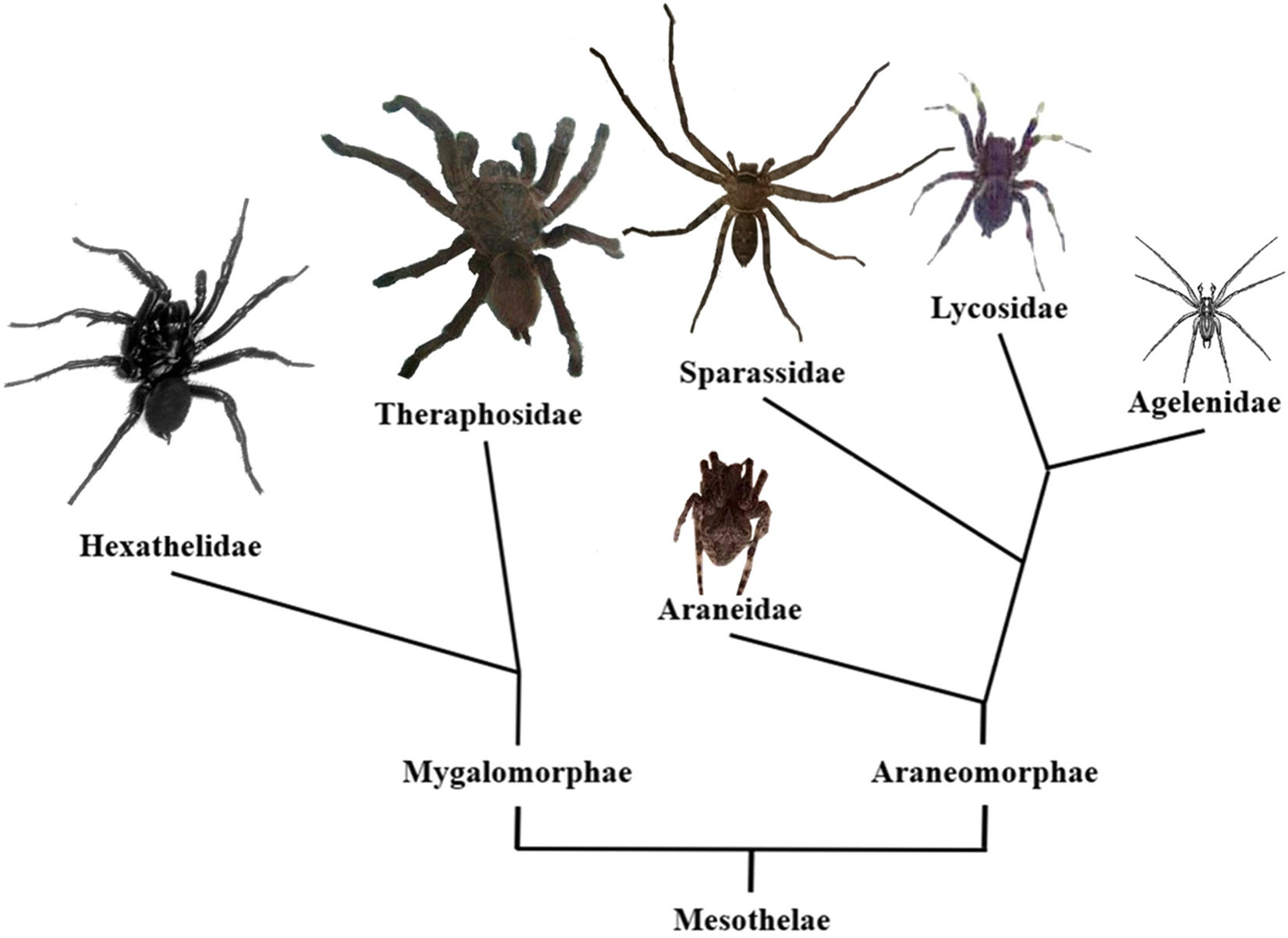This detailed scientific diagram showcases various species of spiders, each represented by either photographs or illustrations, meticulously arranged on a clean white background. The image is structured as a family tree with black lines connecting different species to denote their taxonomic relationships. At the top level, there are central classifications such as Mesothelae, which branches out to Mygalomorphae, further subdividing into families like Hexathelidae, Therophosidae, and Araneomorphae. Additional branches include Lycosidae, Agelenidae, Araneidae, and Mimetidae. Specific examples include a large black spider on the left labeled as Hexathelidae, and a big brown spider to its right identified as Therophosidae, both connecting downward to Mygalomorphae. The spiders are color-coded in hues of black, purple, silver, and brown, with their positions carefully arranged: a central spider placed lower in the diagram, one above it, two in the top right, and two in the top left. This diagram accurately depicts the hierarchical and familial connections among these spider species, providing a detailed and visual taxonomy.